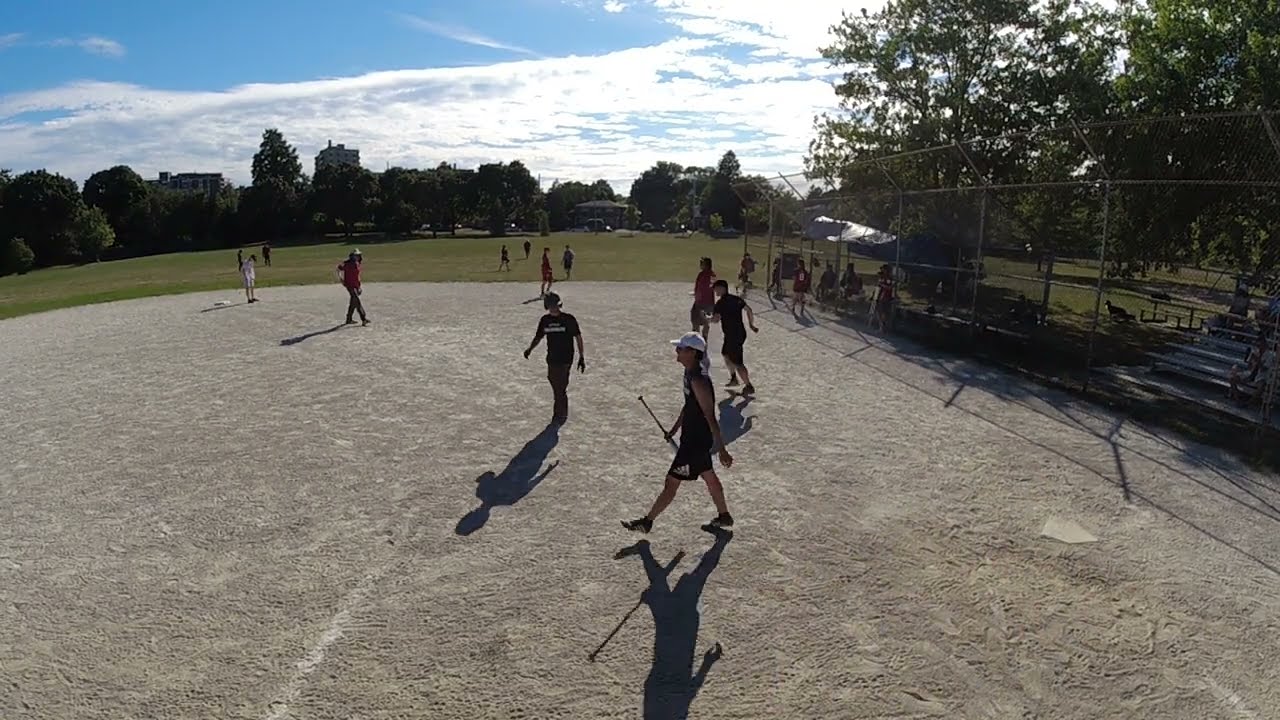In this vibrant photograph taken on a bright sunny day with a blue sky and wispy white clouds, a group of young teenagers are engaged in a casual game of baseball on a well-worn public field. The foreground prominently features the sandy dirt of the baseball diamond, with faded white lines marking areas of play, including a discernible home plate. 

A boy in black shorts, black tennis shoes, a black tank top, and a white baseball cap, standing closest to the camera, holds a baseball bat. Scattered around the field, emphasizing the casual nature of the gathering, are other boys dressed predominantly in black, including in t-shirts and pants, some wearing batting helmets, suggesting that the game has not yet formally started. 

To the right, a tall mesh fence with a bent-inward top borders the field, with bleachers behind it where several people sit, watching the activity. Surrounding the diamond, the lush green outfield stretches into a background of dense trees and residential homes, with tall buildings further in the distance. The scene is lively and picturesque, capturing the essence of a classic day at a neighborhood park.